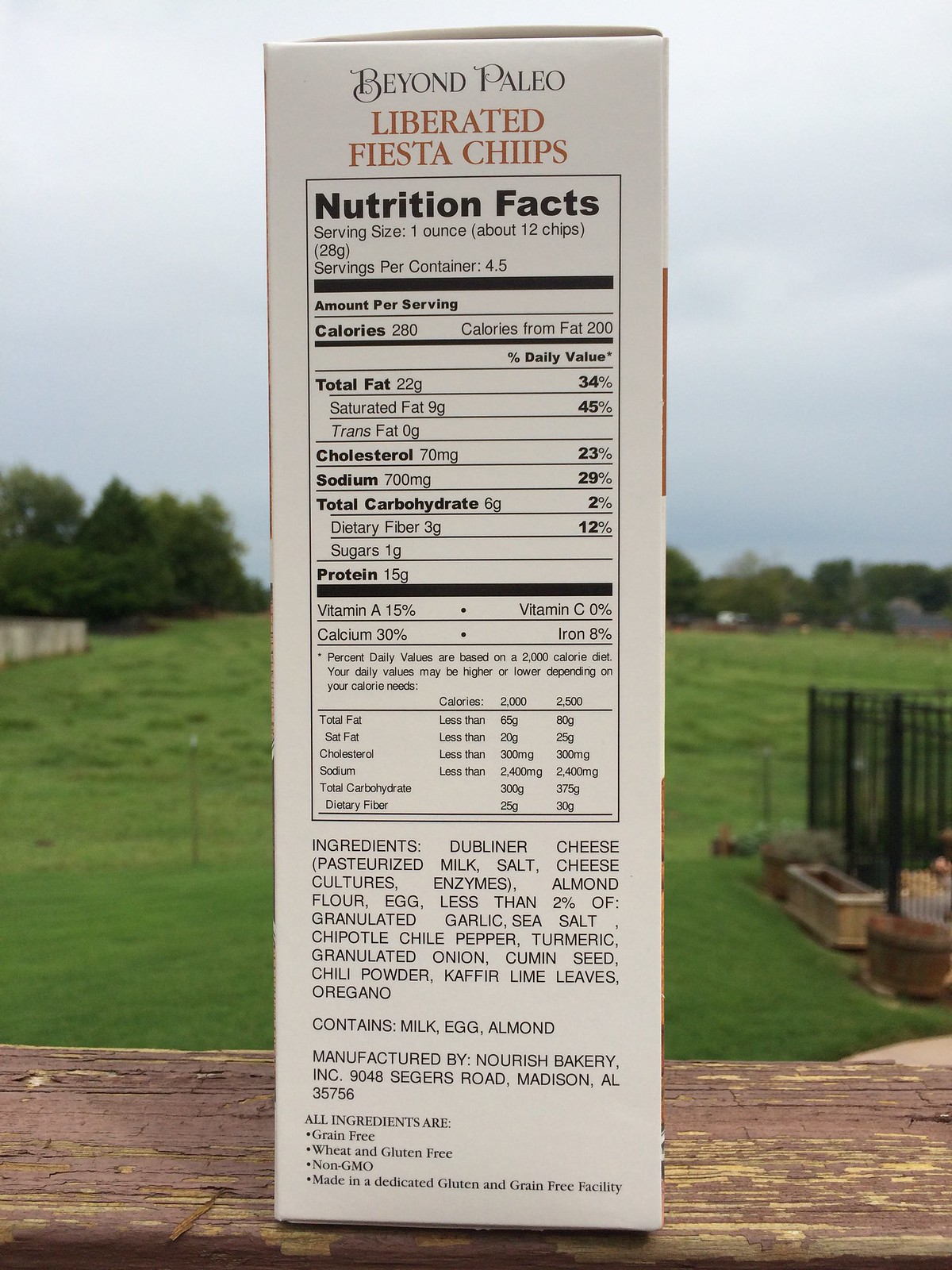In this detailed and descriptive caption, we present an image of a box of chips set on a wooden bench outdoors. The photo's backdrop showcases an expansive open field, punctuated by patches of grass and a scattering of trees in the distance. To the right, a black gate is partially visible, suggesting that the location might be in a park or another open public area.

The focal point of the image is the box of chips prominently placed in the foreground. The box is positioned at an angle, revealing the nutritional information on its side. The brand name, "Beyond Paleo Liberator Fiesta Chips," is clearly displayed.

The nutritional facts are meticulously detailed in black lettering, outlining the serving size, servings per container, and a breakdown of calories, fats, cholesterol, sodium, and carbohydrates. Below this, a comprehensive vitamin section follows. Ingredients are listed in capital letters, emphasizing the product's grain-free, wheat and gluten-free, and non-GMO attributes. It also mentions that the chips are made in a dedicated gluten and grain-free facility. The packaging indicates that the product is manufactured by Norris Bakery, further affirming the health-conscious branding of these chips.